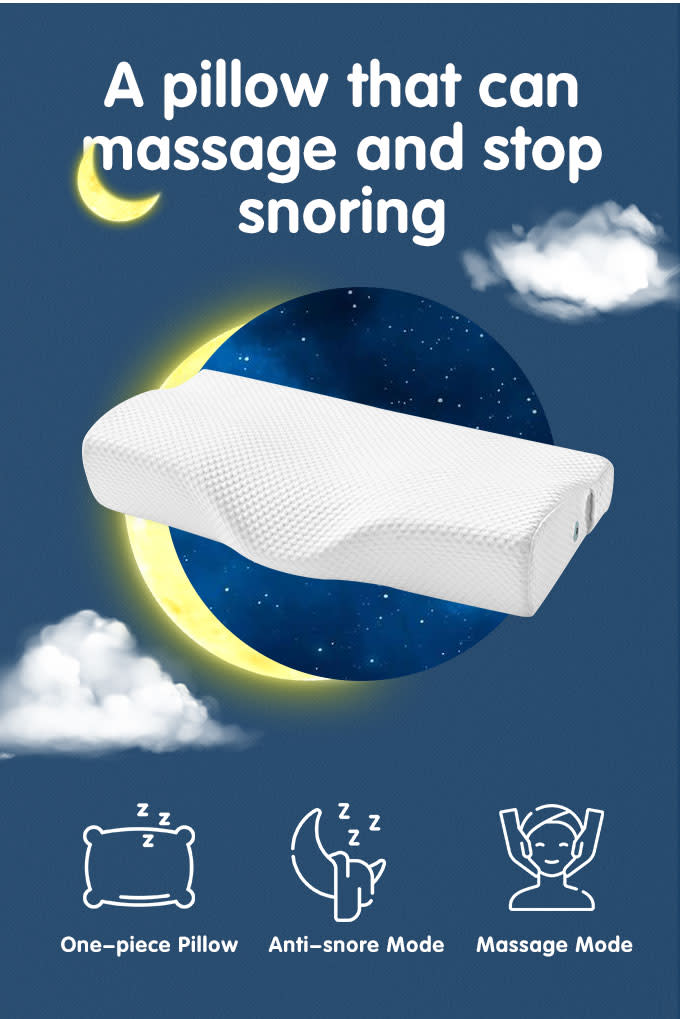This vibrant print advertisement features a revolutionary pillow designed to massage and stop snoring. Set against a medium navy blue, starry background, the ad prominently showcases a white, contoured rectangular pillow with a neck depression, centered on a glowing blue disc with a radiant yellow light. Above the pillow, white text reads, "A pillow that can massage and stop snoring," with a crescent moon hanging from the second line. Fluffy white clouds float gently around the scene, enhancing the serene ambiance. At the bottom of the ad, three illustrations detail the pillow's features: a sketch of the pillow with 'ZZZ' indicating the one-piece construction, a crescent moon draped with a blanket representing anti-snore mode, and an outline of a woman using the pillow in massage mode. The unified design highlights both the innovative functionality and peaceful aesthetic of the product.